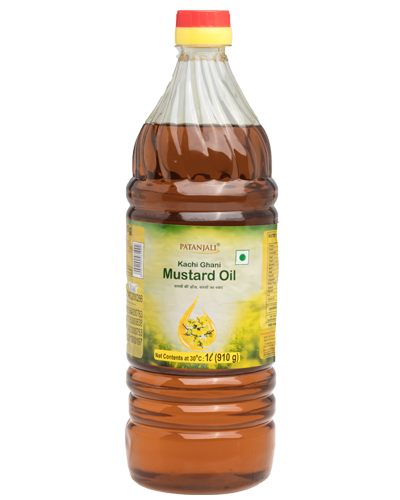The photograph features a single clear plastic bottle prominently positioned against a completely white background, giving it a stock image appearance suitable for online retail. The bottle, partially filled with a brown, tea-colored liquid, sports a two-toned twist cap with red, orange, and yellow stripes. Encircling the bottle is a vividly colored label in green and yellow. The brand name "Patanjali" is written in brown letters, followed by "Kachi Gani" in green, and "Mustard Oil" underneath. Further details in green lettering are too small to decipher. The label also displays a vibrant yellow bouquet of flowers, which adds a decorative element. Additionally, the label indicates that the net content is 910 grams.